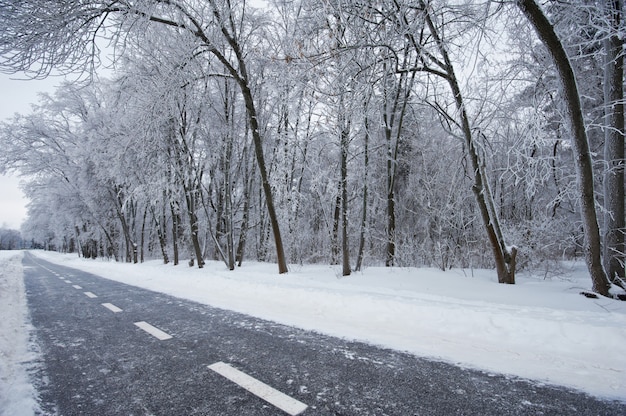This image captures a narrow, single-lane path, likely a bike trail, on a frigid, snowy day. The path, which appears to be made of light gray asphalt, is bordered by thick, solid-packed snow on either side. White lines running down the middle of the path suggest it is meant for cyclists or pedestrians, divided by direction. Surrounding the path are thin, black tree trunks, devoid of leaves, their branches heavy with ice and snow. The entire scene is bathed in a gray, foggy light, with a featureless white sky blending into the background. The overall atmosphere is chilling and desolate, with the pristine snow adding a touch of serenity to the winter landscape.